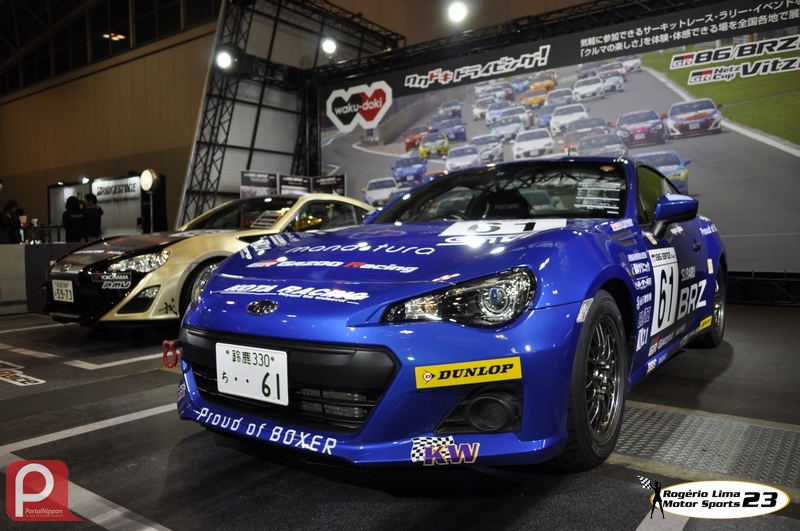The image depicts a showcase room or possibly a display area at a car show, featuring two striking race cars. Dominating the scene is a sleek, shiny purple car with a prominent white number 61 on the driver's side door. This car is adorned with various advertisements, including brands like Dunlop and KW. Notably, the right front fender sports a yellow color, adding a vibrant contrast. Next to it is another race car with a light yellow body and black highlights. Although partially obscured by the purple car, it also displays multiple advertisements. Behind the cars, a large screen shows a live or recorded race, with several cars zooming around a racetrack, enhancing the dynamic atmosphere. The room features parking guide lines on the floor, a red square sign with a white circular letter 'P' in the lower left, and is bathed in colors of purple, tan, red, and white. In the background, there are two people and a round light, suggesting a well-lit, engaging exhibit area that could be in a foreign country, given the non-American alphabet visible at the top.